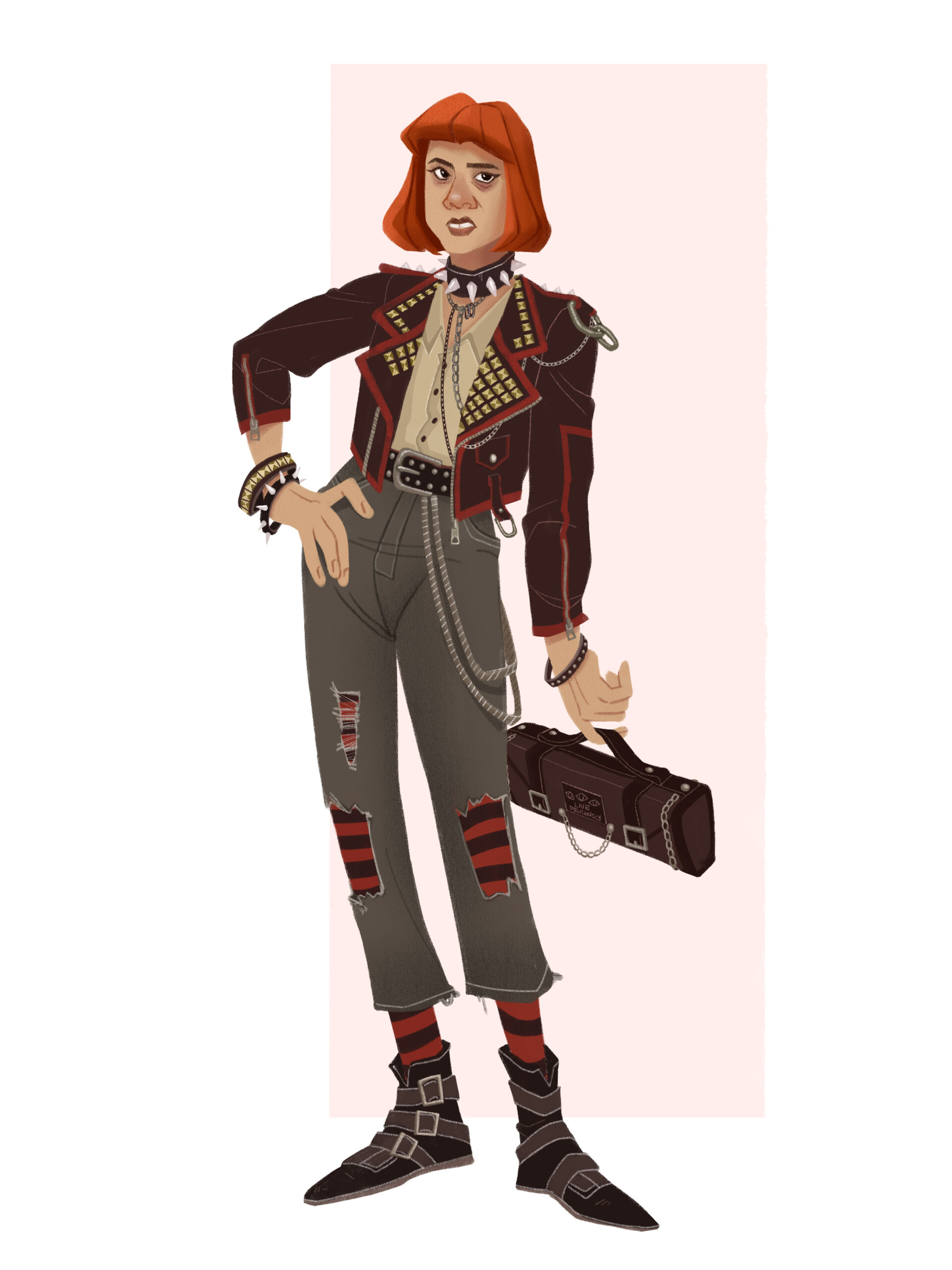The image depicts an androgynous youth with an edgy, punk rock aesthetic, rendered in a cartoon style. The character sports short, red hair styled in a bob and has a look of disdain or sarcasm on their face. They are adorned with a spiked dog collar around their neck and a matching spiked bracelet on their right wrist, which rests on their hip in a nonchalant pose. They wear a black leather jacket reminiscent of Michael Jackson's iconic style, embellished with metal accents and red lines. Their mid-shin length, ripped gray jeans expose red and black striped stockings underneath, which are visible all the way up to their waist through the holes in the pants. Completing the outfit, they have a thick black leather belt with chains, buckle-up boots, and an additional spiked bracelet on their left wrist. The character holds a case in their left hand, which could be interpreted as a black hat purse or an artist's tool set, adding to the image's punk rock, gothic vibe.